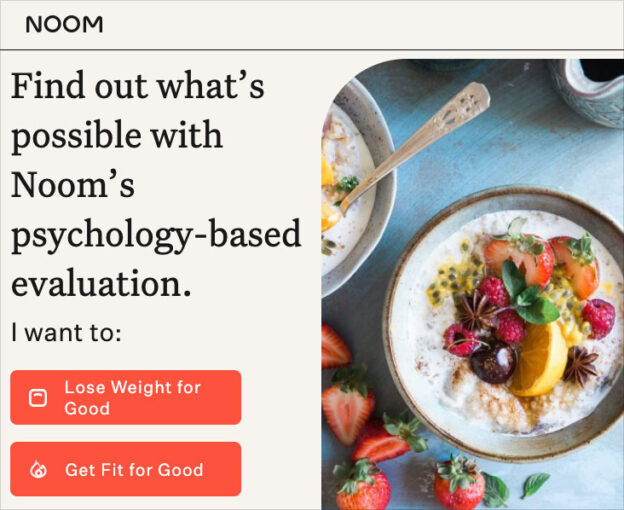This horizontal web page advertisement is for Noom. Positioned in the top left corner, the ad prominently displays the brand name "Noom" in bold lettering, followed by a thin gray horizontal line. The layout of the ad is divided into two sections: text on the left and a photograph on the right.

On the left side, the text is presented in large black font reading, "Find out what's possible with Noom's psychology-based evaluation." Below this, in smaller black text, is the phrase "I want to." Following this are two orange-red horizontal buttons, the first one reading "lose weight for good" and the second one "get fit for good."

The right-hand side features an aerial photograph of a bowl of cereal topped with various fruits, including raspberries, strawberries, and what appears to be segments of an orange. The bowl is surrounded by additional strawberries and partially cut-off by another bowl of cereal at the top left corner of the image. The contents of the bowl appear to be mixed with milk. The photograph is rendered in pastel colors, which complements the ad's overall off-white background and black text for a visually appealing design.